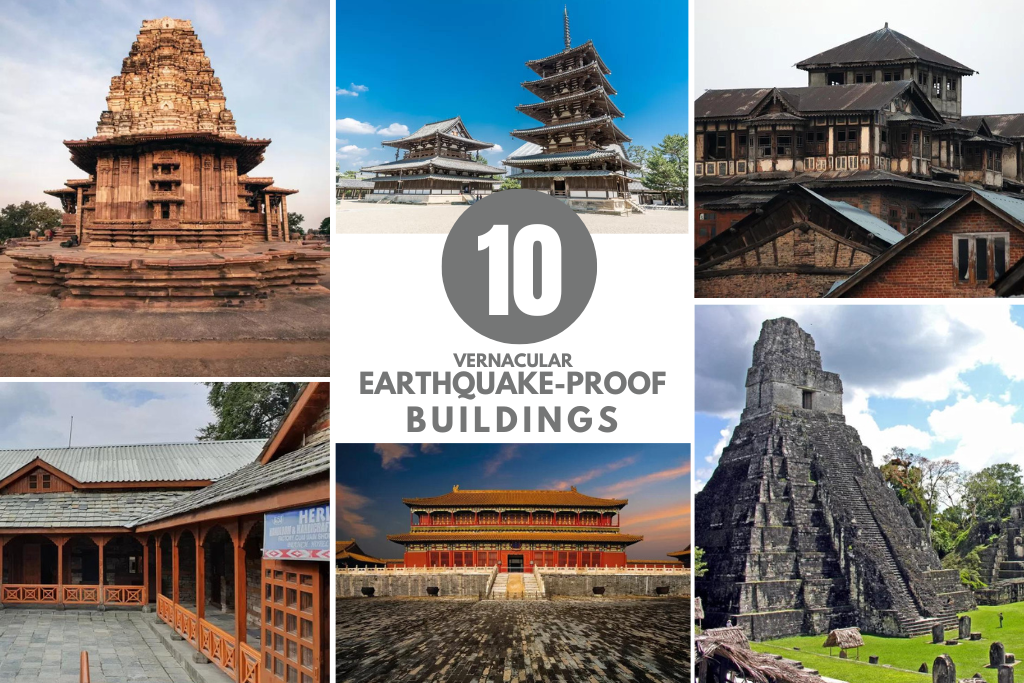The image is a collage resembling a postcard, divided into six sections, each showcasing a different vernacular earthquake-proof building. At the center, there's a gray circle with a white number "10" and beneath it, in gray text, the caption "vernacular earthquake-proof buildings."

- **Top Left**: A brown, hut-style building with barriers in front and a blue sky overhead. 
- **Top Middle**: An Asian-style architecture with gray roofs, designed to withstand earthquakes. 
- **Top Right**: A cluster of dark-colored brick buildings, closely packed together.
- **Bottom Left**: A wooden building nestled among trees.
- **Bottom Middle**: Another Asian-style building, this time with red walls, a brown roof, and steps leading up to it.
- **Bottom Right**: Pyramid-shaped stone structures reminiscent of Mayan ruins, featuring lush green grass and multiple staircases, with possible headstones in the foreground.

All buildings depicted share the theme of traditional architecture engineered to endure seismic activities.